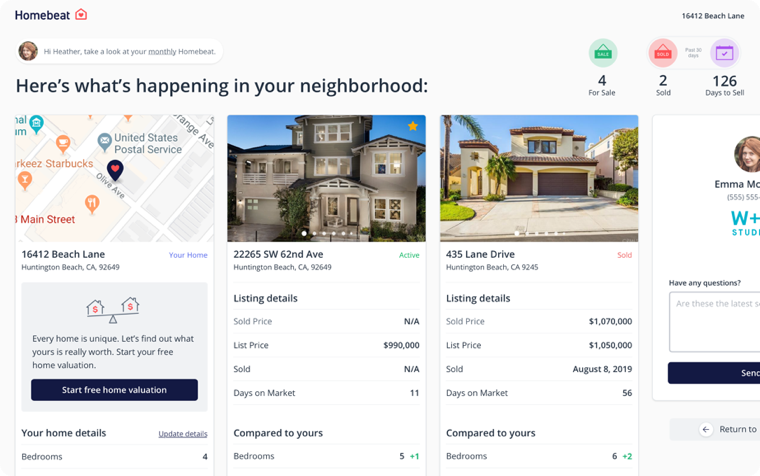The website screenshot showcases a real estate webpage. In the top right corner, the site is branded with the name "Homebeat" accompanied by its logo. On the left side of the image, a section features three colorful icons: a green icon with the label "4 For Sale," a peach icon marked "2 Sold," and a purple icon indicating "126 Days to Sell." Just below this, a prominent header reads, "Here's What's Happening in Your Neighborhood."

The main content area displays three images in a horizontal arrangement. The first image is a detailed map punctuated by multiple pins—colored orange, blue, black, and gray—highlighting various properties. Immediately beneath the map is the address "16412 Beach Lane, Huntington Beach, California, 92649."

Adjacent to the map are two high-quality images of houses. The middle picture features a gray, three-story home designated with the address "22265 Southwest 62 Avenue." The last image showcases a white house with contrasting brown garage doors and roofing, labeled "435 Lane Drive." Each house image includes relevant pricing details and their sale status. Below the address for the property in Huntington Beach is an icon of a scale balancing two houses with red dollar signs, suggesting a pricing comparison.

The overall design is clean and informative, giving a comprehensive view of real estate activity within the specified neighborhood.